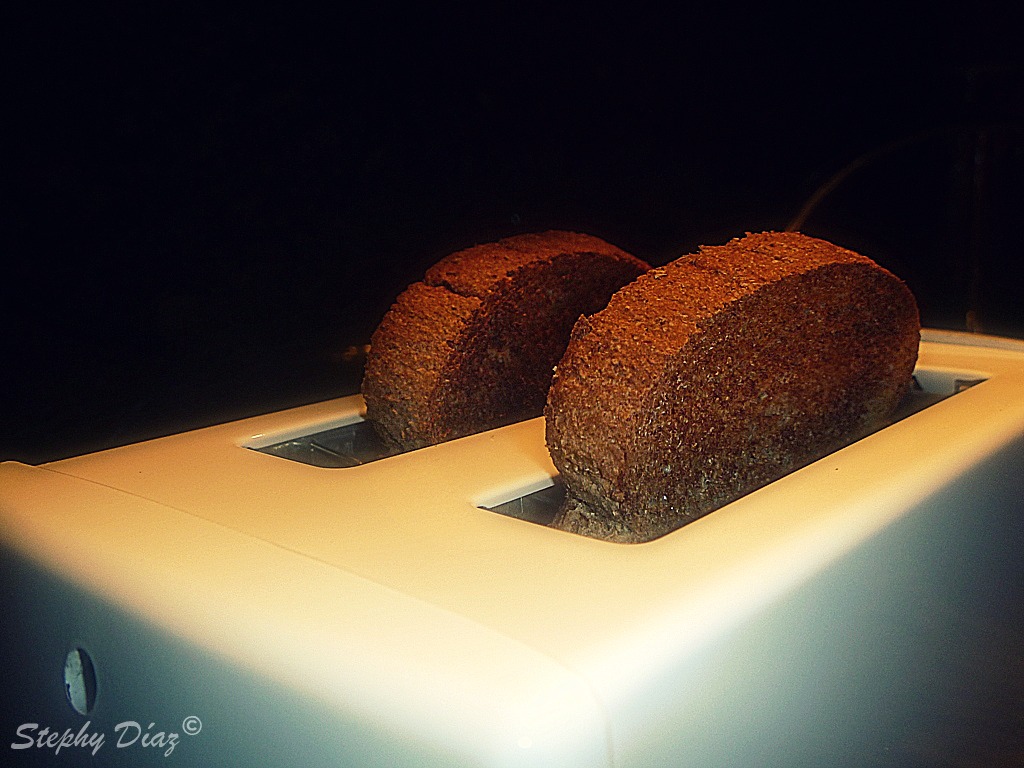The close-up photograph features a white toaster with a thick gray plastic edge on one side. Rising out of the toaster are two thick, dark brown slices of bread, resembling pumpernickel or a health loaf, with a thin crust that's nearly the same color as the interior. Though it's not entirely clear if the bread has been toasted yet, it appears to have the coloring of toasted bread. The backdrop of the image is completely black, obscuring any surrounding environment. In the bottom left corner, the signature "Stephanie Diaz" is visible in a scripted font with a copyright symbol. This watermark highlights the photographer’s name in white cursive, adding an artistic touch to the otherwise straightforward scene. The toaster itself is partially visible, showing mainly the top and a portion of the front without any visible knobs or controls. A small, oval hole can be observed on the short side of the toaster, adding a unique detail.